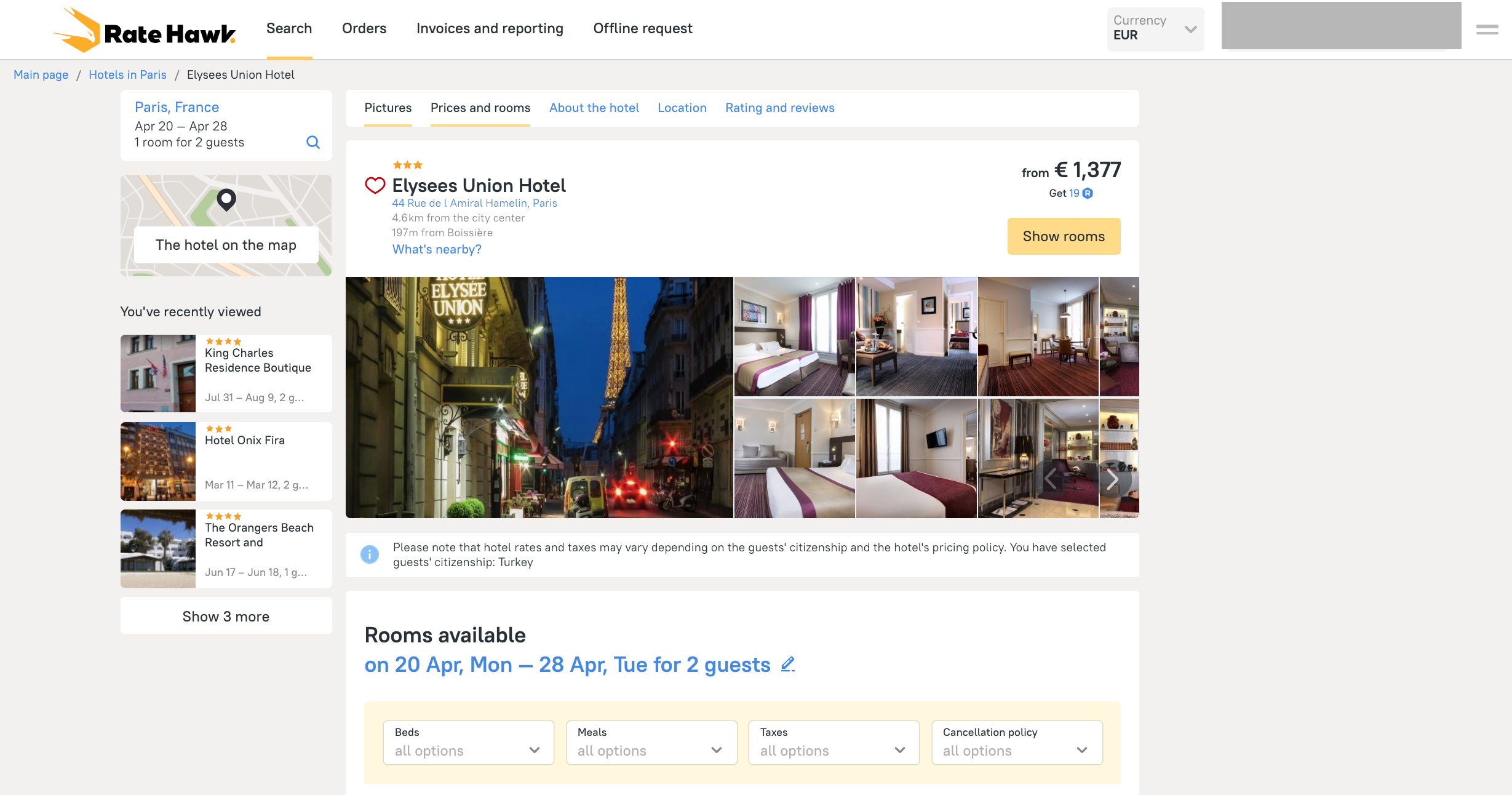The image showcases the RateHawk website with the search section prominently displayed. Users can access various features such as the Order section, Invoices and Reporting section, and Offline Request section. The search section is currently in use, filtered by Euro currency. The main page lists hotels in Paris, and the user is viewing the Elise's Union Hotel, priced from 13.77 Euros per night. The hotel is rated three stars, located 4.6 kilometers from the city center, with options to view nearby attractions and interior photos.

A disclaimer at the bottom advises that hotel rates and taxes may vary based on guest citizenship and hotel pricing policies. The selected guest citizenship is Turkey. The website indicates room availability from Monday, April 20th to Tuesday, April 28th for two guests, with filters for bed types, meals, taxes, and cancellation policies. On the left, the travel details are summarized: Paris, France, from April 20th to April 28th, one room for two guests. The section also shows other recently viewed hotels.